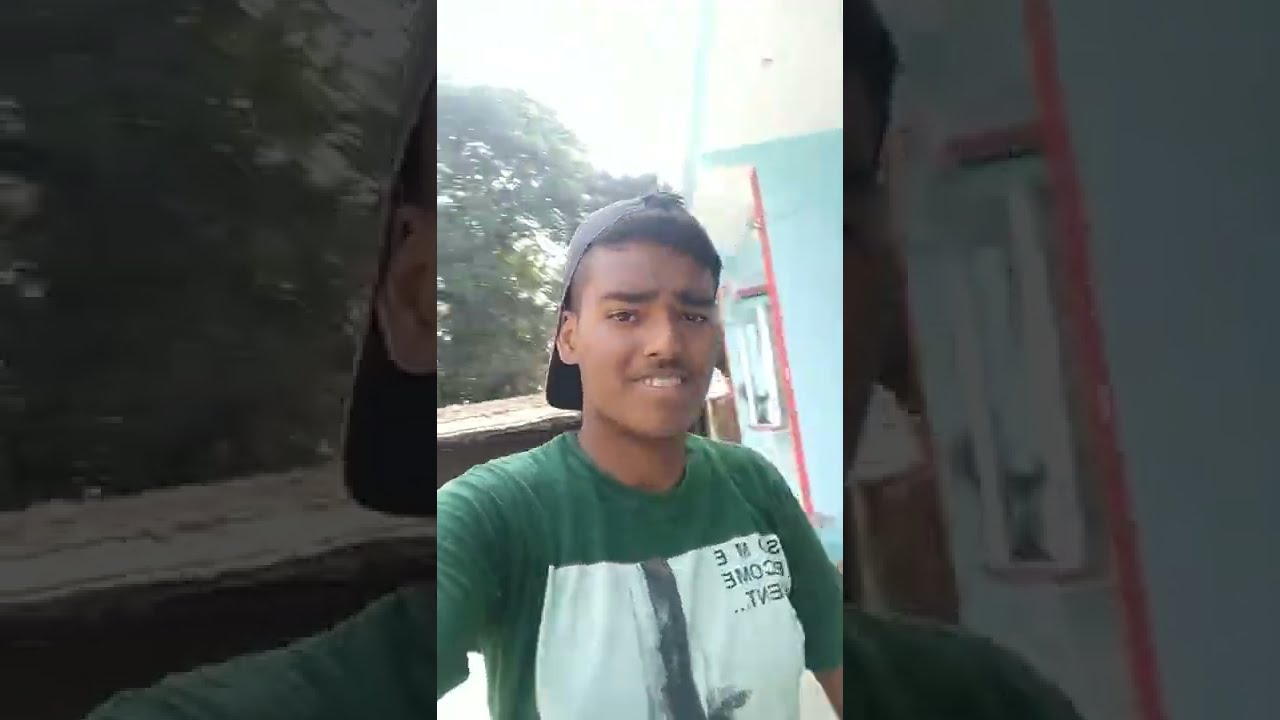This image captures a young man with dark brown, caramel-complexioned skin, and short, cropped black hair, wearing a backwards grey baseball cap. He is seen wearing a dark green, long-sleeved t-shirt with some white and black graphics or text that are not legible due to the angle. The man, who appears to be of Indian descent, is centrally positioned, smiling slightly with a hint of confusion as he looks at the camera, giving the impression that he might be taking a selfie. Behind him, to his left, is a building with light blue walls and red trim, along with a wooden railing. To his right, a tall green tree is visible, adding a natural element to the outdoor setting. The overall quality of the image is not very high, with sunlight casting some highlights that accentuate the scene.